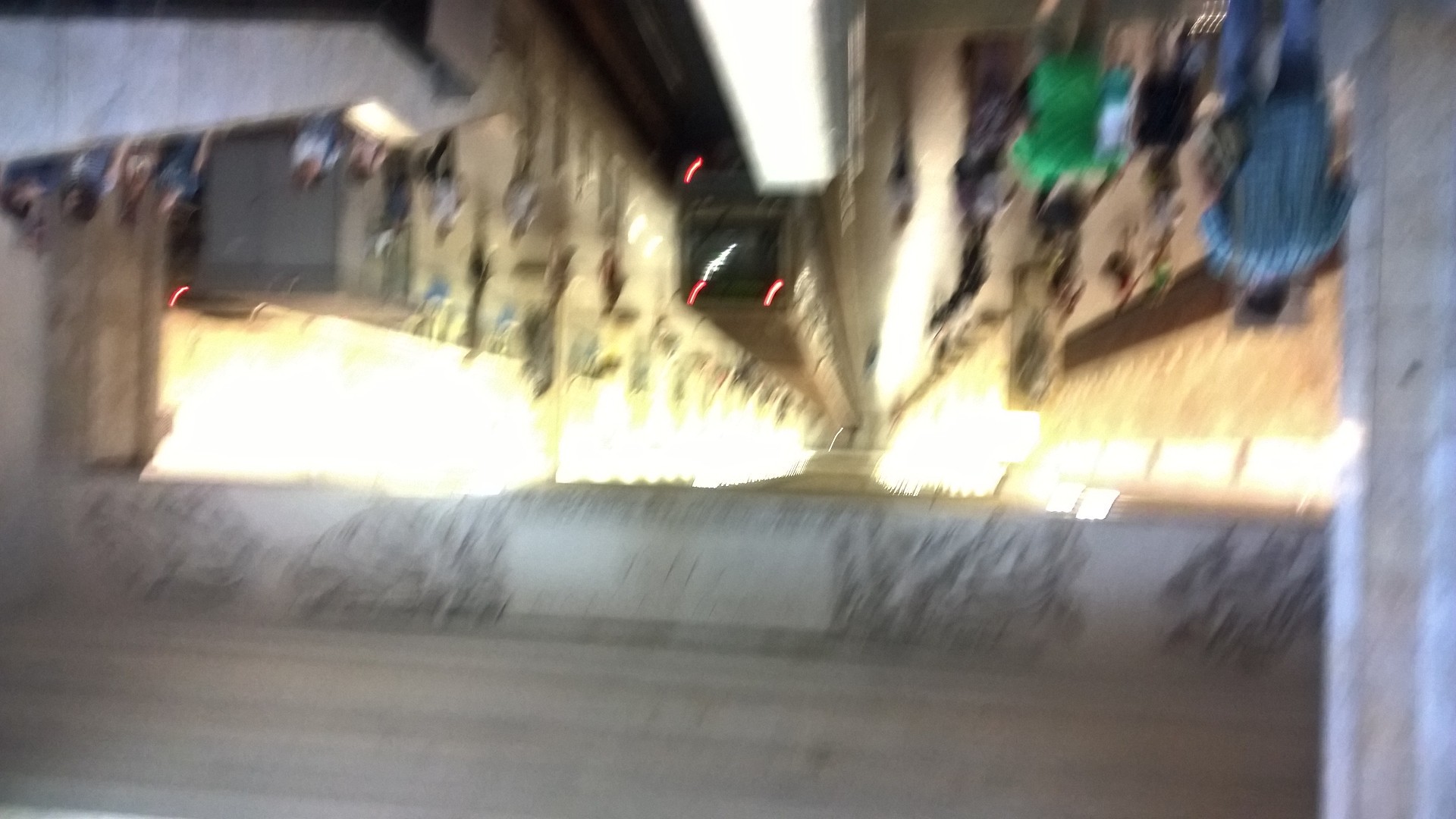The image appears to be inverted, but it depicts a scene reminiscent of a DMV office. On the left side of the picture, a line of people is waiting, possibly for their turn at the service desks. On the right side, customer service representatives are stationed behind their counters. In the center of the room, there is a computer that likely displays wait numbers, although nothing is currently visible on its screen. The ceiling is crafted from white stone with a noticeable pattern; while somewhat out of focus, it features an intricate design of squiggly lines.